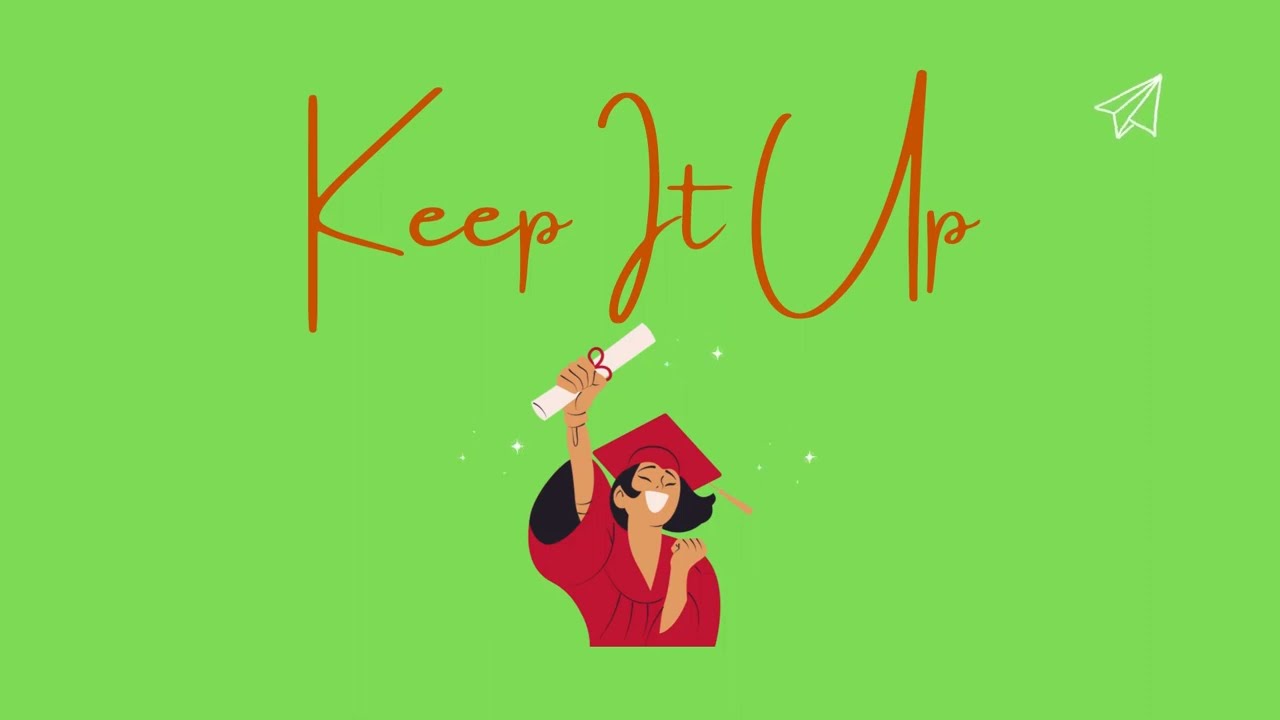Set against a vibrant key lime green background, this image showcases an inspiring scene. In the upper right corner, a white paper airplane adds a whimsical touch. At the top center, the motivational message "Keep it up" appears in large, red script-like letters. Below this text, a celebratory figure dominates the scene: a cartoon graduate with brown skin, wavy black hair, and a beaming white smile. She is adorned in a red graduation gown with a black interior and a matching red cap featuring a tassel. Her right hand triumphantly holds up a white diploma wrapped with a red ribbon, while her left hand is clenched in a victorious fist. This image encapsulates the joyful culmination of academic achievement and encourages perseverance and continued success.